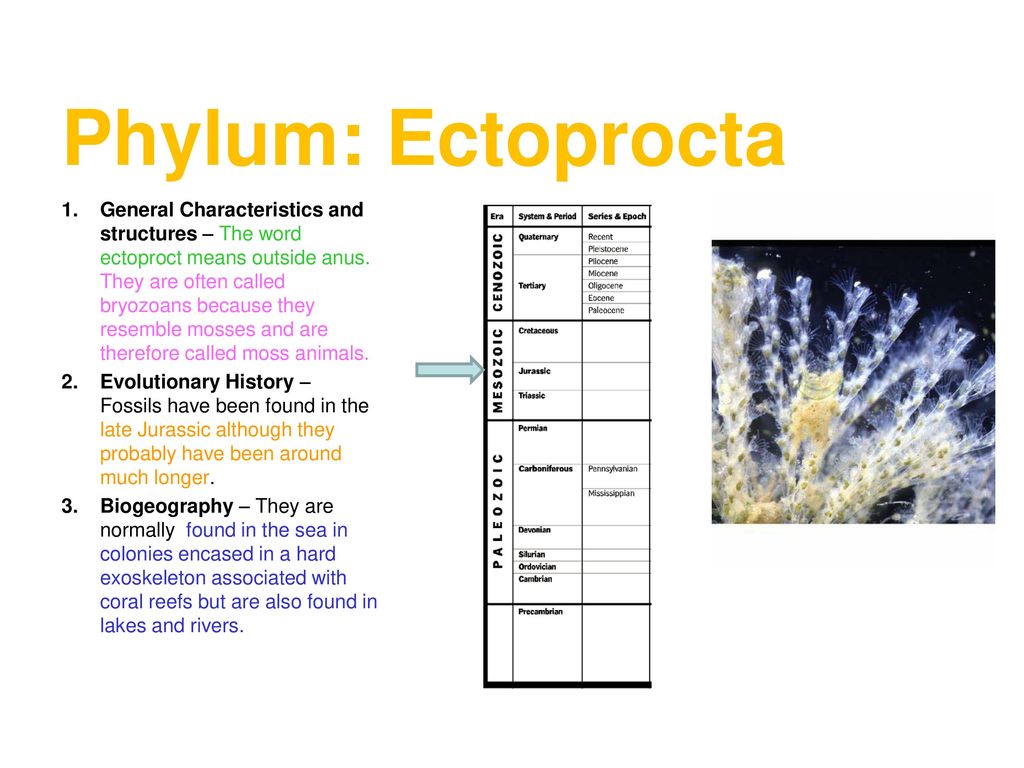The image is an educational reference, likely from a biology textbook or PowerPoint slide, detailing the phylum Ectoprocta. The content is set against a white background, with a bold, large headline in golden yellow reading "Phylum: Ectoprocta." Below the title, there are three numbered bullet points describing general characteristics and structures, evolutionary history, and biogeography, each in various text colors.

1. **General Characteristics and Structures:** The first bullet point explains that "ectoproct" means "outside anus," with the text in green and purple. It further details that these organisms are often called bryozoans because they resemble mosses and are commonly known as moss animals.
   
2. **Evolutionary History:** The second bullet, a mixture of black and gold, notes that fossils of ectoprocts have been found from the Late Jurassic period, although it is likely they have existed for much longer.
   
3. **Biogeography:** The third point, in black and blue, describes that ectoprocts are usually found in the sea, forming colonies within hard exoskeletons associated with coral reefs, but they can also be found in freshwater environments like lakes and rivers.

To the right of the bullet points, there is a chart that categorizes time periods into eras, systems, periods, series, and epochs, with a pale blue arrow pointing specifically to the Mesozoic era. Below the chart, a close-up photograph of ectoprocta showcases their delicate, translucent structure, resembling a coral reef with lightly fanned, spine-like projections dotted along their lengths, forming a cluster within a watery environment.

Overall, the image is designed for educational purposes, using a streamlined and colorful layout to convey detailed information about ectoprocta in a clear and accessible manner.